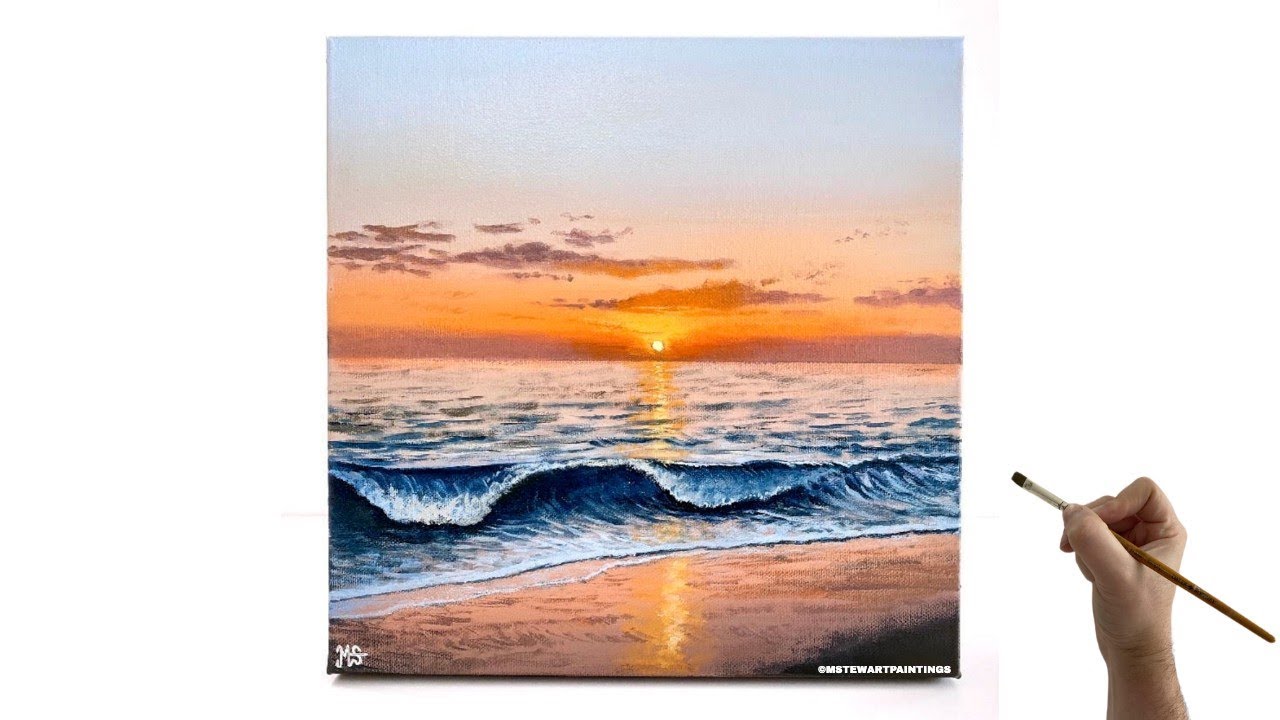The image depicts a perfectly square painting of a serene ocean scene at sunset, framed against a white background. The ocean is a rich blue, with waves cresting a few feet behind a sandy beach that bears footprints in the sand. A narrow path of golden light from the setting sun stretches across the water to the shore. The sky is a gradient of radiant oranges and deepening blues, adorned with purple clouds. To the right of the painting, a Caucasian hand holding a thin paintbrush extends just below the wrist, suggesting the presence of the artist. The painting is meticulously signed with "M-STEWART paintings" in the bottom right corner, and the initials "M-S" on the far left. The entire composition hints at a realistic yet slightly digital feel, adding a modern touch to the classic seascape.